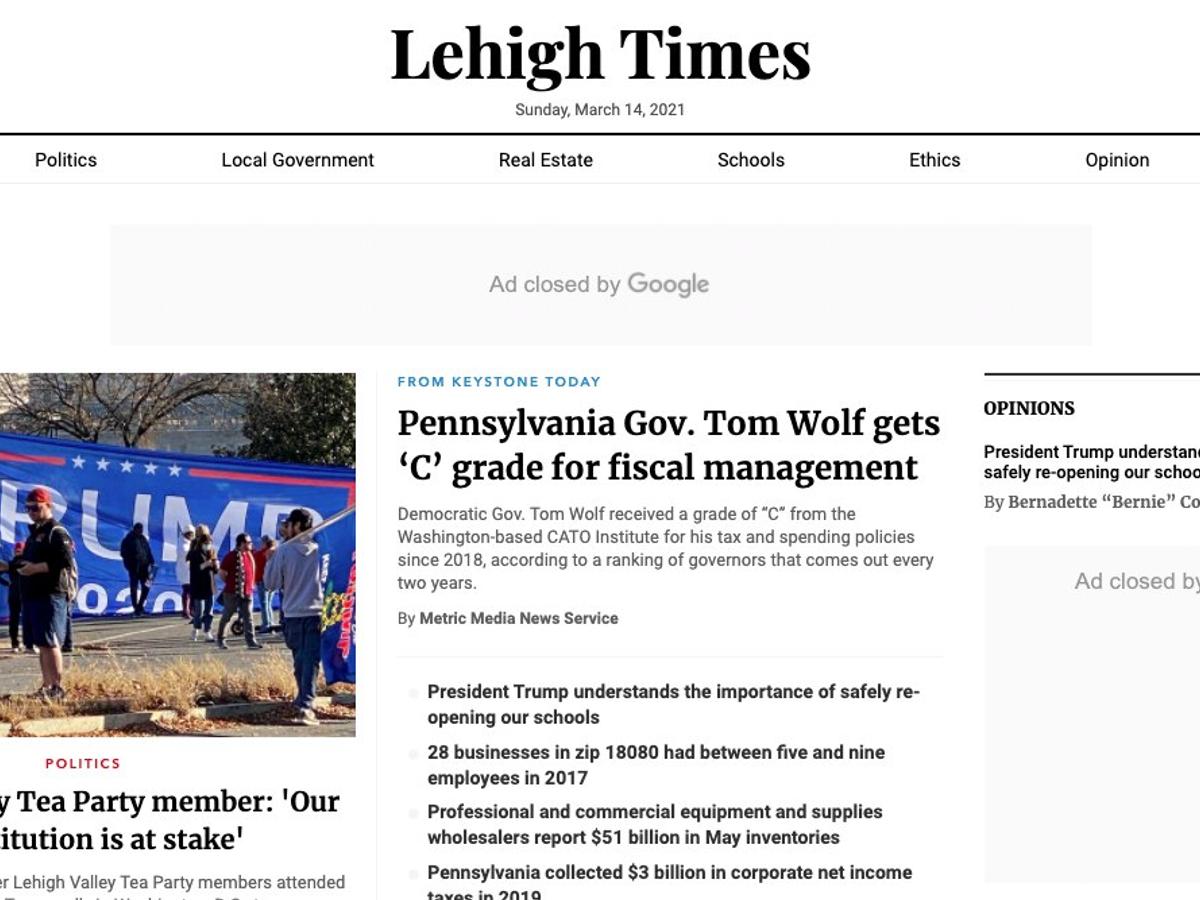This image features the main screen of an online newspaper, "Lehigh Times," dated Sunday, March 14, 2021. The header is clearly marked with the newspaper's title and date, followed by a black line that delineates the various sections of the publication. The navigation bar includes categories such as Politics, Local Governments, Real Estate, Schools, Ethics, and Opinions. Below these sections, there is a gray box containing the text "ad closed by Google."

Prominently displayed is a headline from "Keystone Today" featuring the main article: "Pennsylvania Governor Tom Wolf Gets C Grade for Fiscal Management." The article details that Democratic Governor Tom Wolf received a C grade from the Washington-based Cato Institute for his tax and spending policies since 2018, according to a biannual ranking by Metric Media News Service.

On the left side of the screen is an image depicting a political scene with a large Trump flag in the background, indicating a likely connection to Trump supporters or Tea Party members.

Beneath the main article, clickable headlines for additional news stories are listed, including:
- "President Trump Understands the Importance of Safely Reopening Our Schools."
- "28 Businesses in ZIP Code 18080 Had Between Five and Nine Employees in 2017."
- "Professional and Commercial Equipment and Supplies Wholesalers Report $51 Billion in May Inventories."
- "Pennsylvania Collected $3 Billion in Corporate Net Income Taxes in 2019."

On the right-hand side of the screen, there is a dedicated section for opinions, rounding out the layout of the newspaper's main interface.